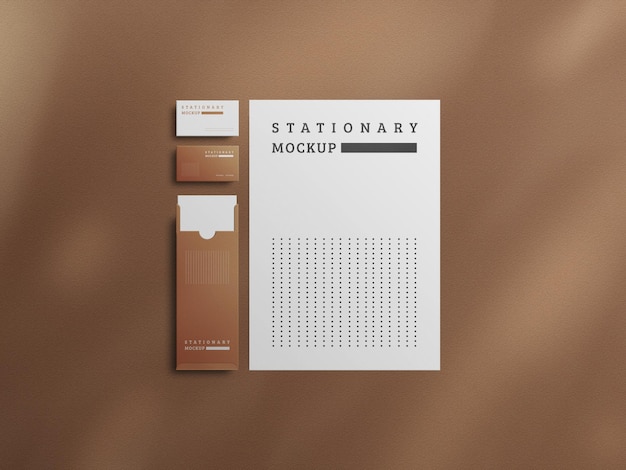This detailed image showcases a stationery mock-up against a mostly brown background. Centered on a brown wall, the focal point is a standard piece of white paper with "Stationery Mock-up" text written across the top. Below this title, a little black bar is followed by a blank area, and the bottom half of the page is marked with evenly spaced dots. To the left of the paper are two business cards; the top card is white with brown text, while the card beneath it is brown with white text. Below these cards is an elongated brown envelope featuring the text "Stationery Mock-up" in white. The scene also includes a small cardboard box with white pieces of paper in it, positioned to the left of the main sheet. The overall color palette prominently features shades of brown, white, and tan, emphasizing a professional, stock image vibe for showcasing business paper products.